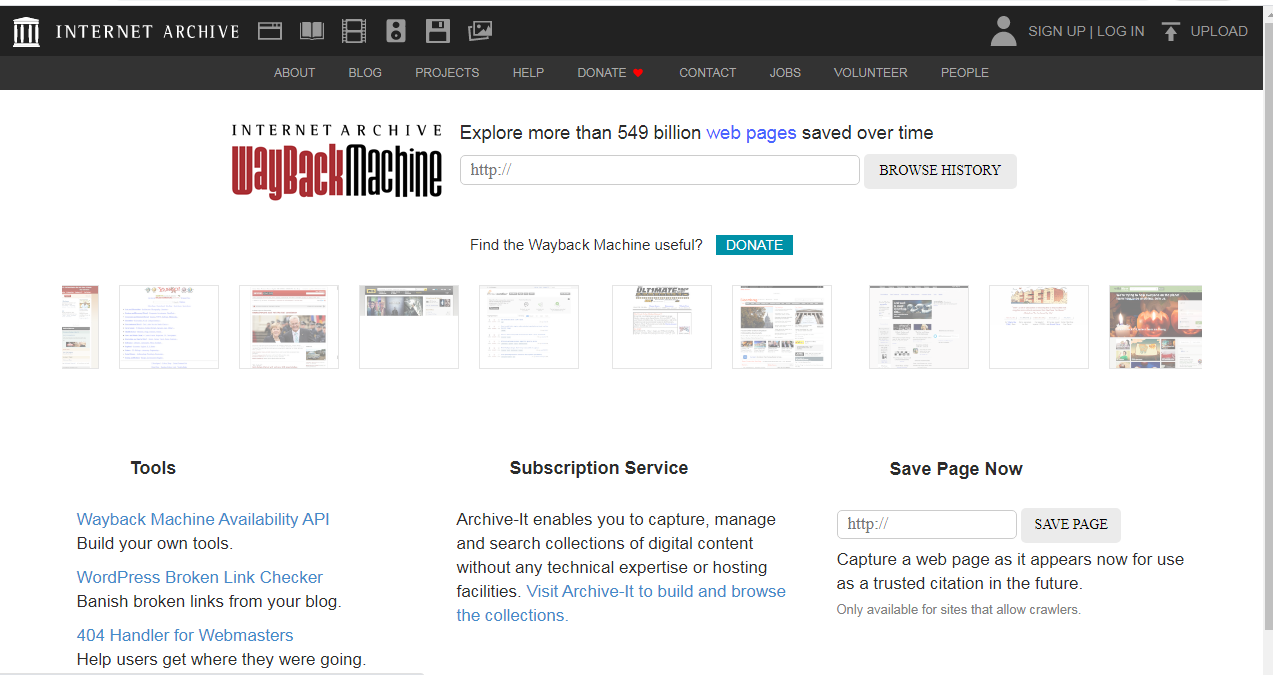Here we have an image depicting the homepage of the Internet Archive. At the top of the page, there is a horizontal black bar featuring the Internet Archive logo, which resembles books on a shelf, accompanied by the text "Internet Archive" in white. To the right of the logo, there are various icons representing different types of media: books, videos, audio, floppy disks, and images.

In the top right corner, there are buttons for signing up, logging in, and uploading content. Directly below the black bar, there are tabs for navigating to sections such as About, Blog, Projects, Help, Donate, Contact, Jobs, and Volunteer.

The main content area has a white background and prominently displays the heading "Internet Archive Wayback Machine," highlighting that it has explored and saved over 59 billion web pages over time. Below this heading, there is a search bar to enter URLs and browse the web history.

Further down, there is a prompt reading "Find the Wayback Machine useful?" with a "Donate" button positioned to the right. Following this section, various images are displayed.

At the bottom of the page, there are three distinct sections: the first labeled "TOOLS" with related options, the center section titled "Subscription Service," and the third section "Save a Page Now," which includes a box to enter a web link to save it.